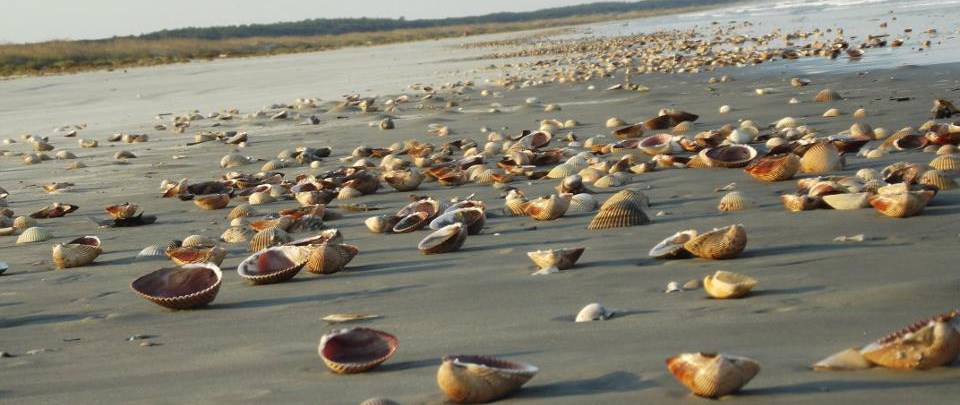In this wide-angle, full-color photograph taken outdoors during the daytime, the focal point is a beach littered with hundreds of half-shells, likely clamshells, washed ashore and arranged in a natural wave pattern. The shells, predominantly brownish in color, are all tipped up on their backs, creating a textured foreground against wet, grayish-beige sand. No footprints disturb the sand, suggesting minimal human presence.

In the top right corner, water can be seen crashing onto the shore, indicating the tide's influence in depositing these shells. Beyond the beach, the horizon features a light green field transitioning to darker green trees, adding a natural backdrop to the scene. The photograph is rectangular and captures this marine life setting without any borders, text, or people, emphasizing the serene, undisturbed quality of this coastal landscape.